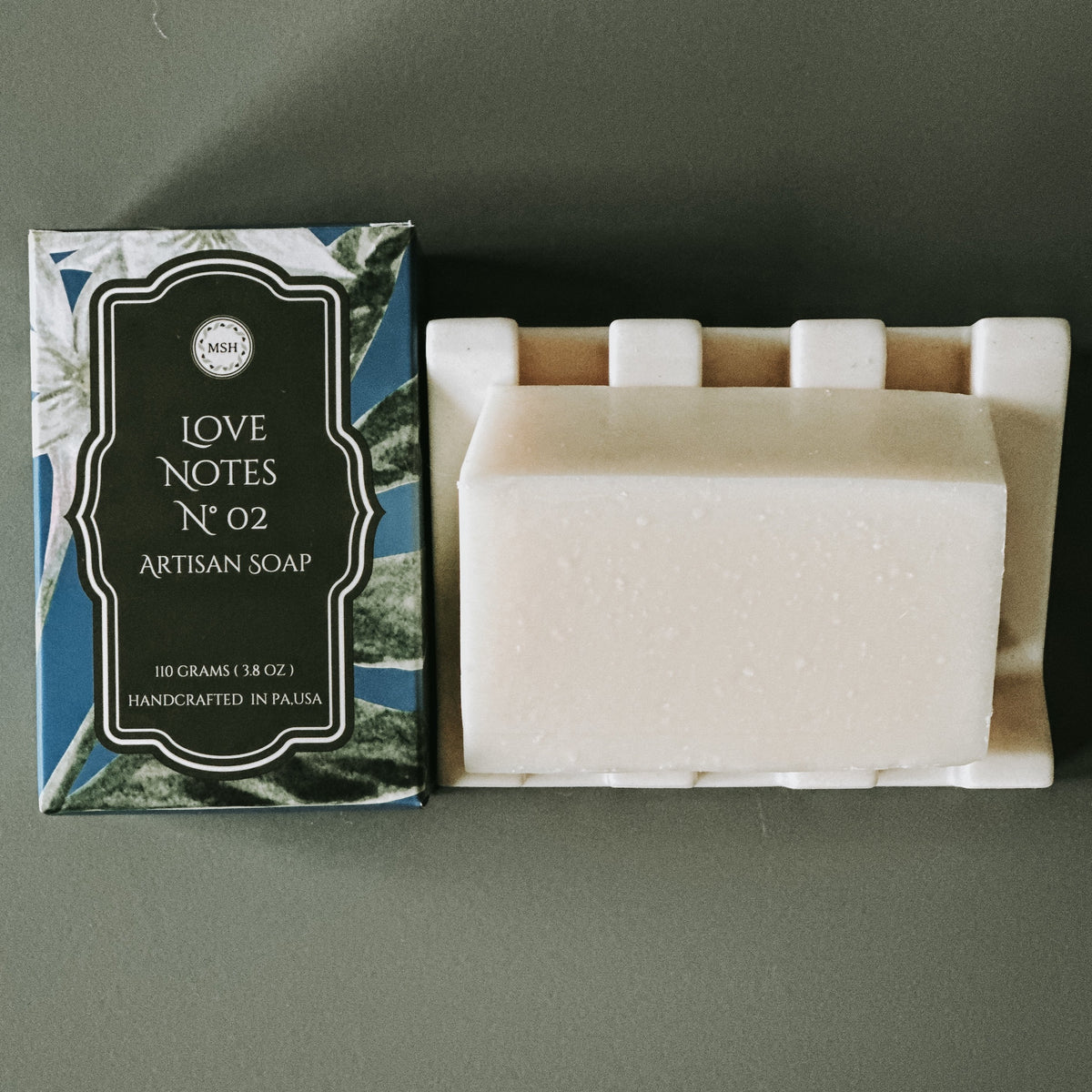This is a detailed photograph featuring a bar of Love Notes No. 2 Artisan Soap from MSH, along with its ornate packaging. The soap, a pale almond white color with visible crevices, rests on a white soap display dish on the right-hand side. The packaging, situated on the left, is an elaborate paper design boasting a black insignia-like sign with white lettering against a backdrop of green leaves and white flowers on a blue background. The package clearly states "Love Notes No. 2 Artisan Soap, 110 grams (3.8 ounces), handcrafted in Pennsylvania, USA." The entire scene is set against a dark gray background, emphasizing the artisanal and handcrafted elements of the product.